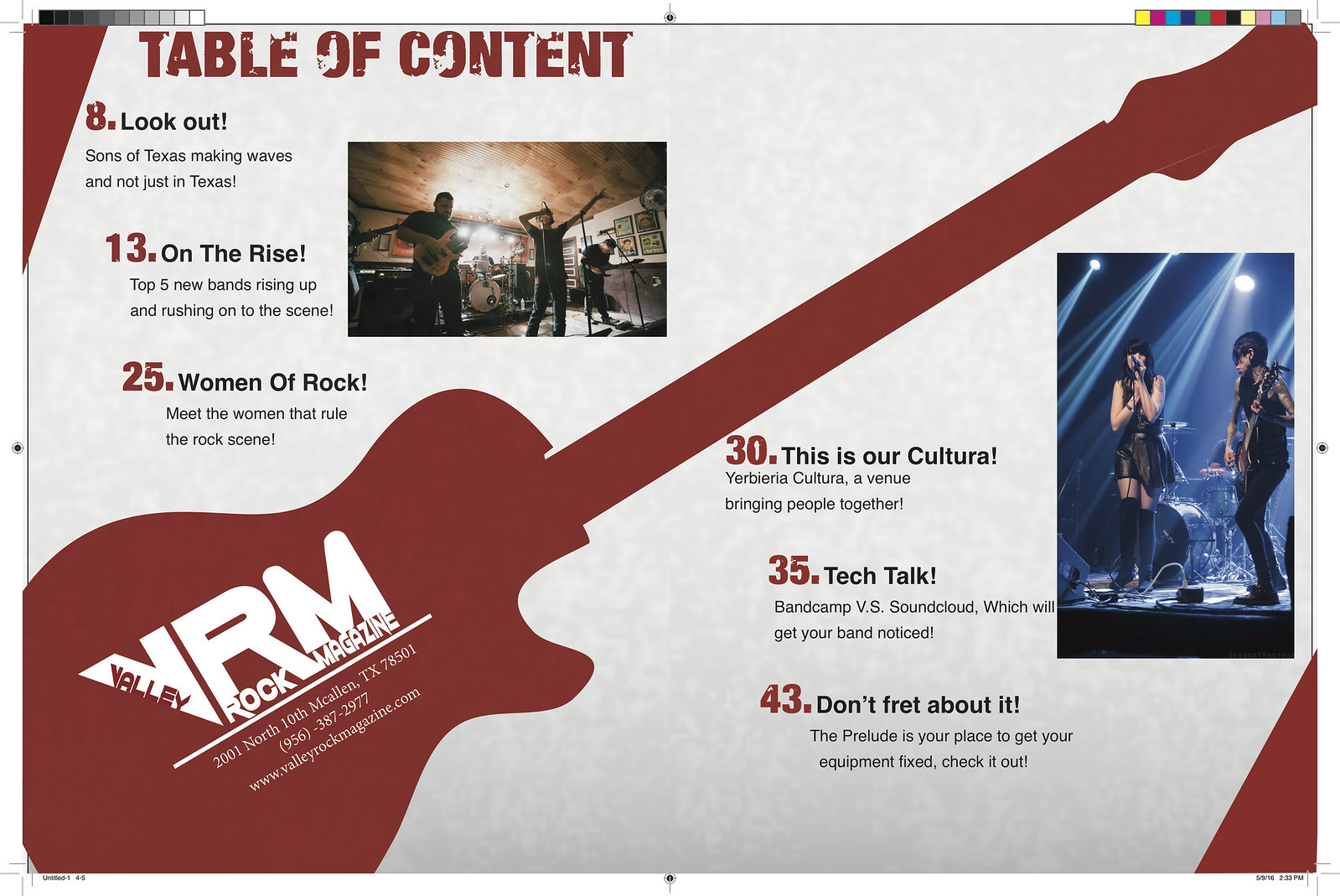This image portrays an open rock magazine featuring a detailed table of contents spread across two pages. At the top left corner, the heading "Table of Content" is prominently displayed. The layout is artistically designed with red and black text, interspersed with red highlights, providing a visually striking contrast. Dominating the spread, a red-outlined guitar diagonally stretches from the lower left side of the first page to the upper right corner of the second page, creating a seamless visual bridge between the pages.

On the table of contents, key articles are listed with page numbers in red, followed by titles in black text. Key features include: "8 Look Out - Sons of Texas making waves," "13 On The Rise," "25 Women of Rock - Meet the women that rule the rock scene," "35 Tech Talk - BandCamp versus SoundCloud: Which will get your band noticed," and "43 Don’t Fret About It - The prelude is your place to get your equipment fixed."

The spread is further enriched with two photographs of rock acts and a collection of bold colors including off-white, yellow, orange, brown, and blue. Additionally, the magazine details "Valley VRM Rock Magazine 2001 North 10th, McAllen, Texas" within the guitar outline, enhancing the promotional flair of the piece. This dynamic blend of images and text epitomizes the magazine's rock essence, engaging readers with its vivid and organized presentation.